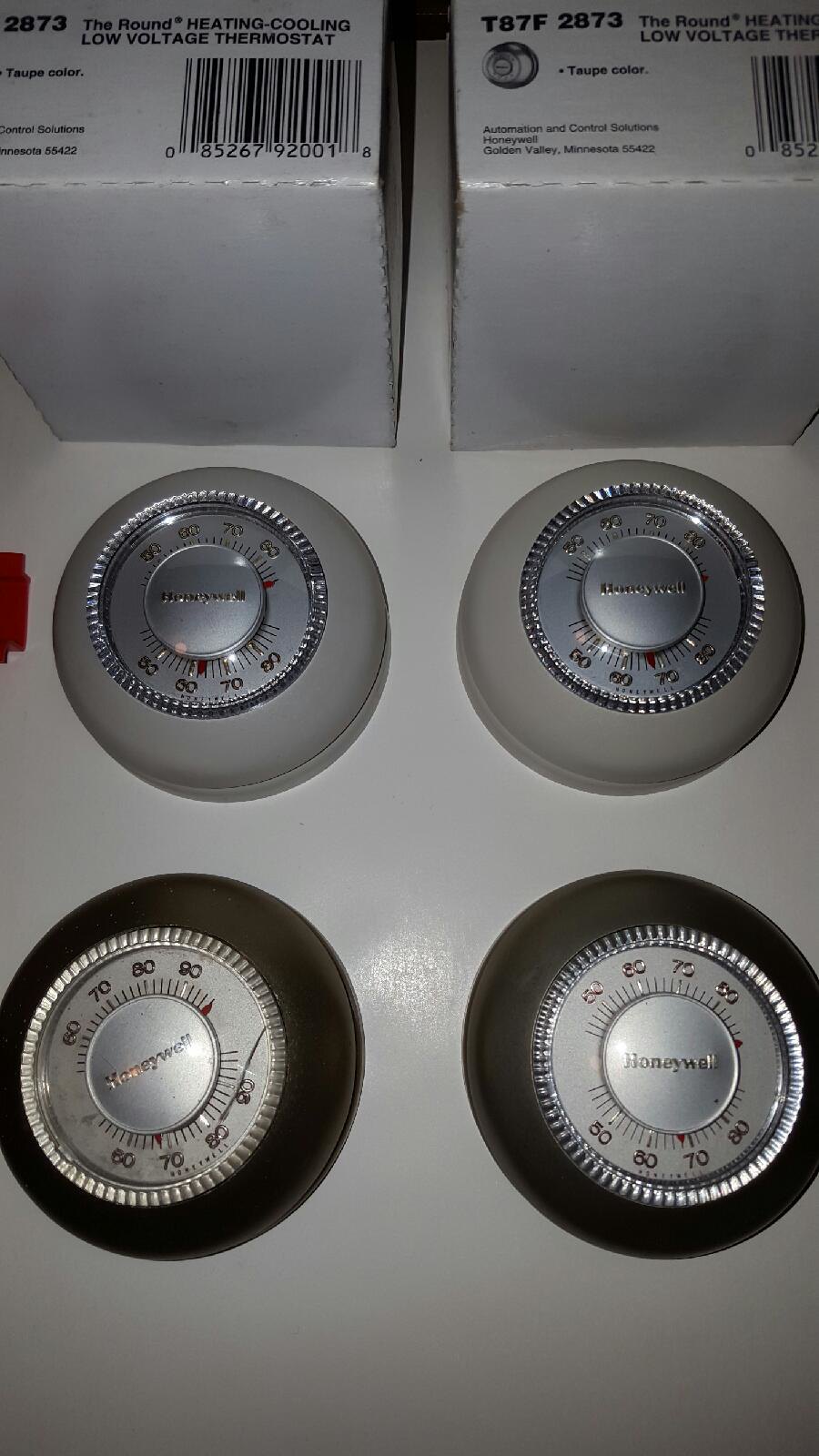This image captures a top-down view of four thermostats arranged in two rows, accompanied by their packaging. At the top of the image, there are two white boxes with barcodes, each labeled with "The Round Heating Cooling Low Voltage Thermostat," indicating a taupe color. Additionally, the boxes bear the inscription "Automation and Control Solutions Honeywell, Golden Valley, Minnesota 55422." 

Below these boxes, four Honeywell thermostats are lined up. The two at the top are light gray and bear the Honeywell logo in the middle. Although the numbers are somewhat difficult to read, the temperature scale on these units appears to range from 50 to 80 degrees Fahrenheit. 

The two thermostats on the bottom row are darker, with a brownish-dark gray hue, and also feature the Honeywell name centrally placed. The temperature scales on these bottom units are more legible, showing increments of 60, 70, 80, and 90 degrees Fahrenheit.